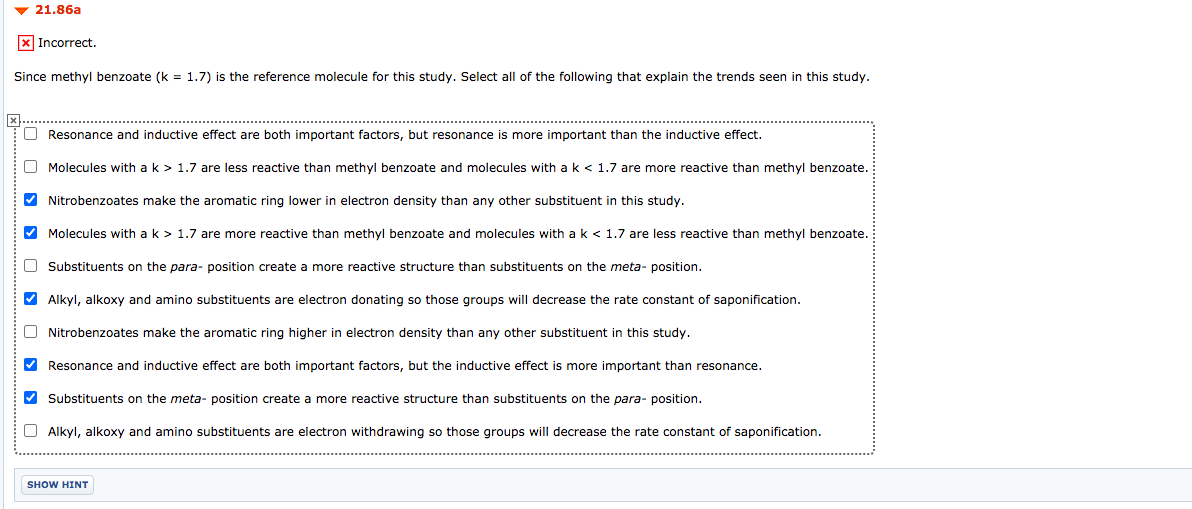The image displays a webpage with a highlighted red header at the top, prominently featuring the value "21.86". On the left side of this header, there is a red downward-pointing arrow. Below this, in black text, it states the information is incorrect, accompanied by a red box containing a red "X". 

The page mentions "since methanol benzoate" and indicates that "K equals 1.7" is the reference molecule for the study. It then prompts the user to select all relevant explanations for the trend observed in the study. 

There is another distinct section outlined with black dotted lines, almost resembling a cut-outable area. Within this section, there is a comprehensive list of categories, each represented by boxes. Some of these boxes are white, while others are filled blue with a white check mark. The categories include terms like "resonance", "inductive effect", "molecules on nitro benzoate", "substituents on the para position", "alkyl", "aloxy nitro benzoates", "resonance inductive effect substituents", "alkaloids", "aloxy", and "amino substituents".

At the bottom of the image, there is a "Show Hint" button, suggesting that users can click it for additional assistance if needed.